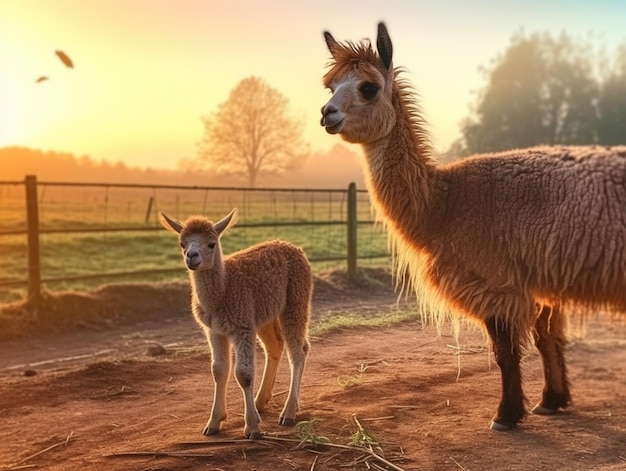The photograph captures a serene scene featuring an adult llama and a baby llama standing on a dirt road, both gazing towards the camera. The mother llama, standing on the right with a thick tan coat, seems alert, her ears rimmed in black and pricked up attentively. The baby llama, positioned to the left in front of her, appears more serene, oblivious to its surroundings. Both animals have shaggy brown fur with grayish-white faces and a reddish-brown tuft of fur between their ears. Surrounding them is a wooden fence with three horizontal railings and wire between the posts. Beyond the fence lies a grassy area with scattered dead grass and a prominent tree. In the background, the sun sets to the left, casting a warm, golden glow over the entire scene and illuminating a distant hillside adorned with trees and bushes. A paraglider can be seen in the sky, adding a touch of adventure to the tranquil setting.